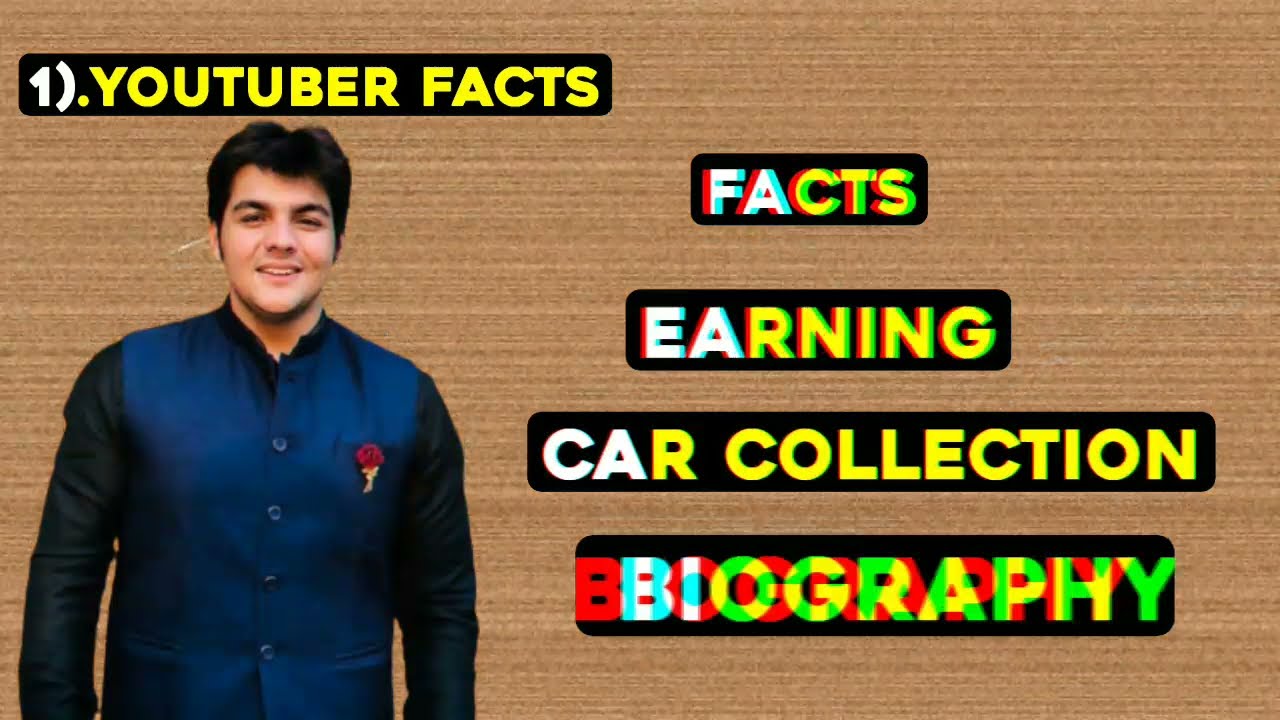The image appears to be a YouTube thumbnail or an advertisement, prominently featuring a young man in his early 20s to late 20s with dark hair and a reddish complexion. He is smiling, displaying the top row of his teeth, and looking directly at the camera. He is dressed in a blue button-up jacket, resembling a uniform, with a red rose logo on the left breast pocket and long black sleeves. 

The background of the image is a symmetrical, faux wood grain texture, digitally inserted through green screen technology. At the top of the image, there is text in white letters stating "Number One," followed by "YouTuber Facts" in yellow text. To the right of the man, a series of words are listed vertically: "FACTS," "EARNING," "CAR COLLECTION," and "BIOGRAPHY." These words are rendered in a mix of white, yellow, red, and green text, with each word appearing on its own black background. Notably, the word "BIOGRAPHY" is displayed in an overlapping, double-vision style with letters in alternating colors of white, green, and red.